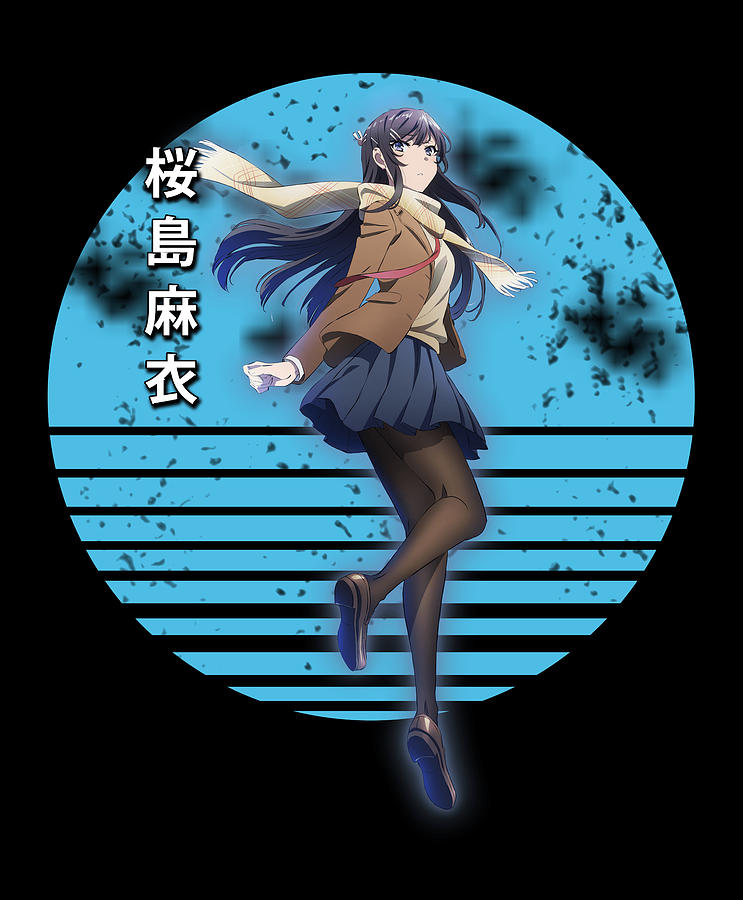This illustration depicts a dynamic manga-style female character set against a predominantly black background. Central to the art is a large blue circle, adorned with black specks and segmented black lines growing thicker towards the bottom. To the left of the circle, four vertical Asian kanji characters descend in a line. The character, occupying the center of the illustration, has long, dark hair reaching down her back with bangs, and she appears to be jumping or turning mid-air, as she lifts one leg. Her attire includes a short, pleated navy blue skirt, black tights, black flat shoes, a brown blazer over a beige shirt, and a beige and white scarf. She faces slightly to the right, poised elegantly in this visually striking composition.